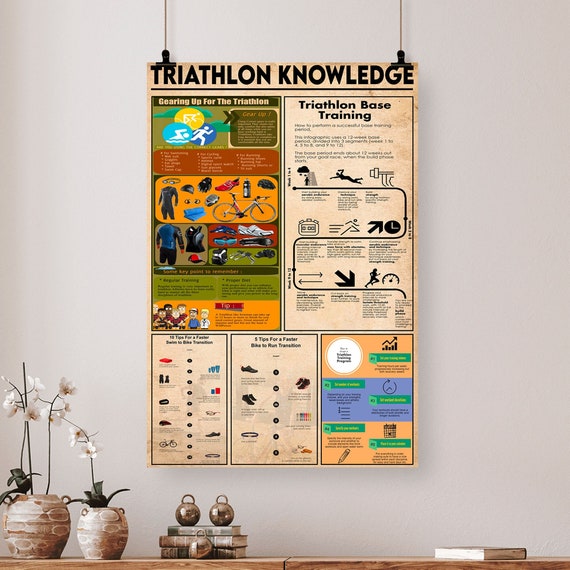This photograph captures a neat and well-organized interior space, likely a study or living area, featuring a prominent poster hanging from two strings affixed by black clips against a white wall. The poster, titled "Triathlon Knowledge" in bold black letters, serves as an informative chart about triathlons, depicting illustrations and text on topics such as bicycling, swimming, equipment, and techniques. The lower portion of the image reveals the top edge of a brown wooden shelf or table. Situated on this surface are two tan ceramic vases holding orchid flowers, with one vase slightly taller than the other. Alongside the vases is a neat arrangement of books: three stacked books with metal paperweights on top, and a single book resting to the far right.